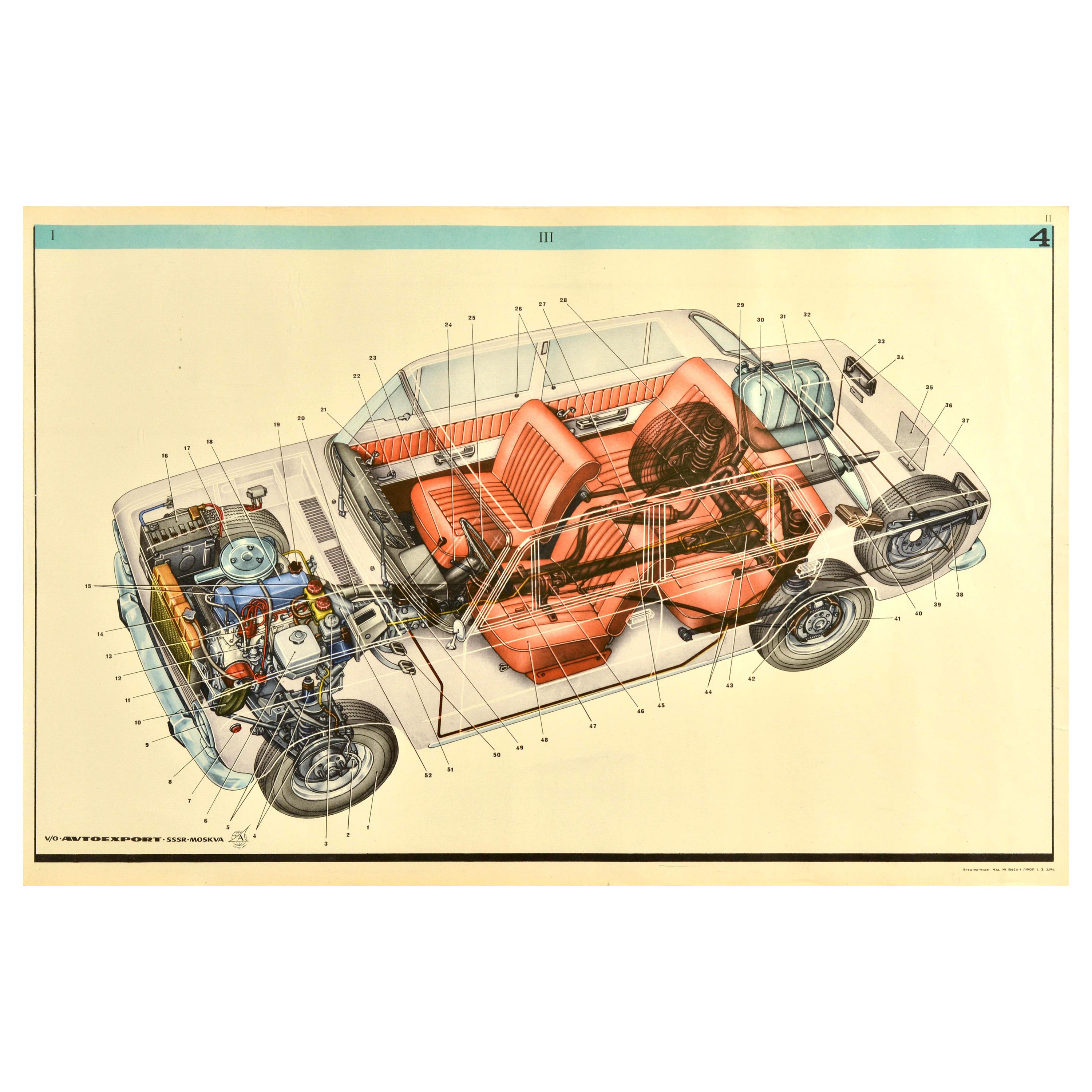The image depicts a detailed schematic drawing of a sedan vehicle, presented on yellowish, light-colored paper. The drawing offers a top-down view of the car, with the front of the vehicle positioned in the lower left and the rear in the upper right. Significant parts of the interior and exterior are visible and labeled with numbers, though the key to these numbers is not included on the diagram.

The car's structure is clearly outlined, revealing components such as the orange or reddish-colored seats, the engine in the front, and the trunk area in the back which includes a spare tire and an additional compartment. Elements such as the wheels, axles, and the gas tank are also discernible.

The paper features a thin green or teal border at the top with a number in the middle that may be "1H" and a bold "4" in the right corner. In the bottom left corner, the text "Auto Export SSR Moskva" is written just above a black line, with additional small, unreadable writing in the bottom right corner beneath the border. The overall schematic is well-lit, making the car’s components clearly visible despite the small and somewhat blurred text.